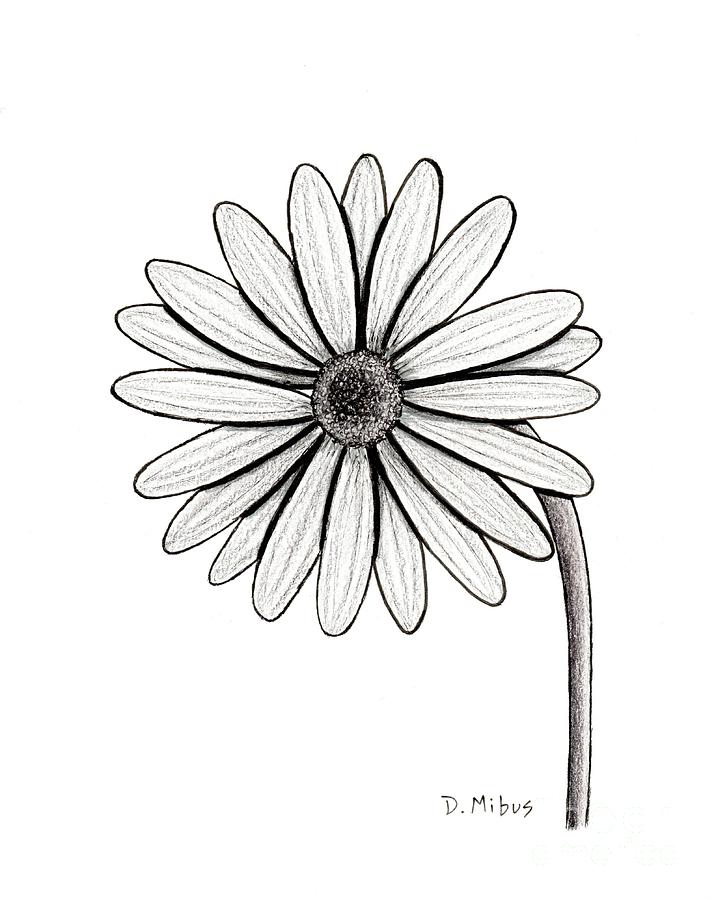The image depicts a black and white drawing on an entirely white background, blending seamlessly without visible edges. The artwork features a large flower that resembles a daisy or sunflower, characterized by its dark round center and numerous light, thin, long petals that fan outwards. There is notable shading within the petals and along the stem, which starts at the bottom right, curves slightly to the left, and extends upward. At the bottom right corner of the image, the artist's signature, "D. MIBUS," is handwritten in black letters, with the "D" and "M" capitalized.